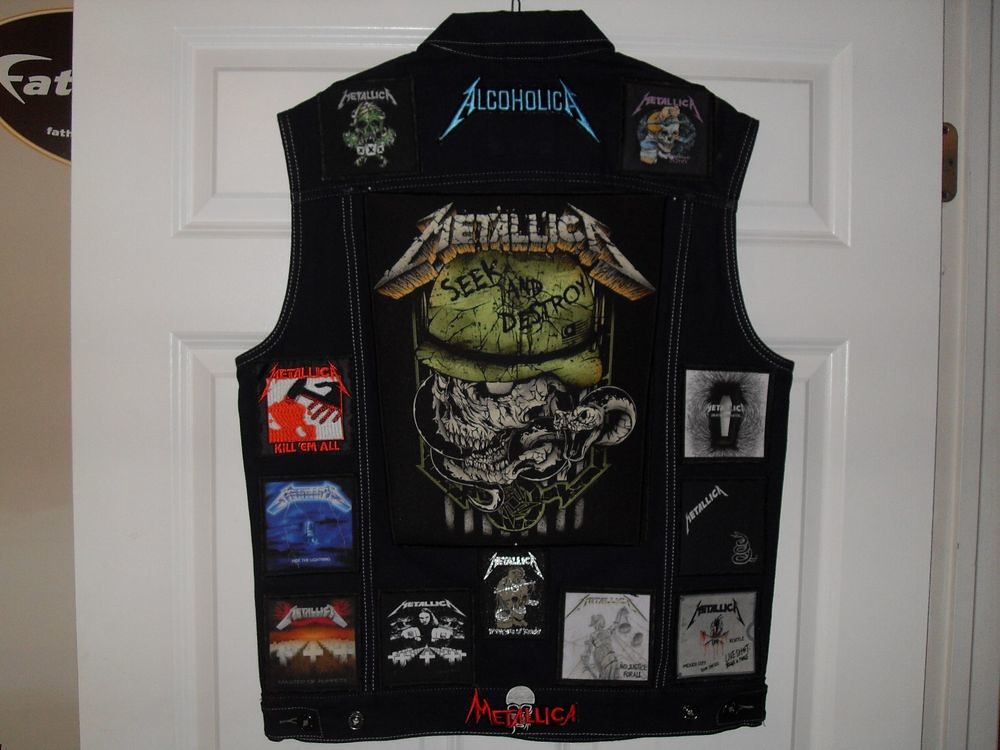This image depicts the back view of a black, sleeveless jean vest hanging on a white door via a hanger. The vest is adorned with numerous patches and text primarily related to the band Metallica. Dominating the center is a large patch featuring a skull and a snake, with the iconic band name "Metallica" written across it in red. Above this central patch, at the top of the vest, the word "Alcoholica" is prominently displayed. Additional smaller patches are scattered across the vest, showcasing various images such as hammers, skulls, and possibly other band logos, all contributing to a heavily customized and rugged aesthetic. The setting of the photograph is indoors, with a beige wall partly visible behind the door. An oval-shaped sign with partly legible letters "F.A.T." can be seen to the left of the door, adding a bit more context to the room's decor. The photograph is horizontally aligned, capturing the vest in detail against the contrasting white door.